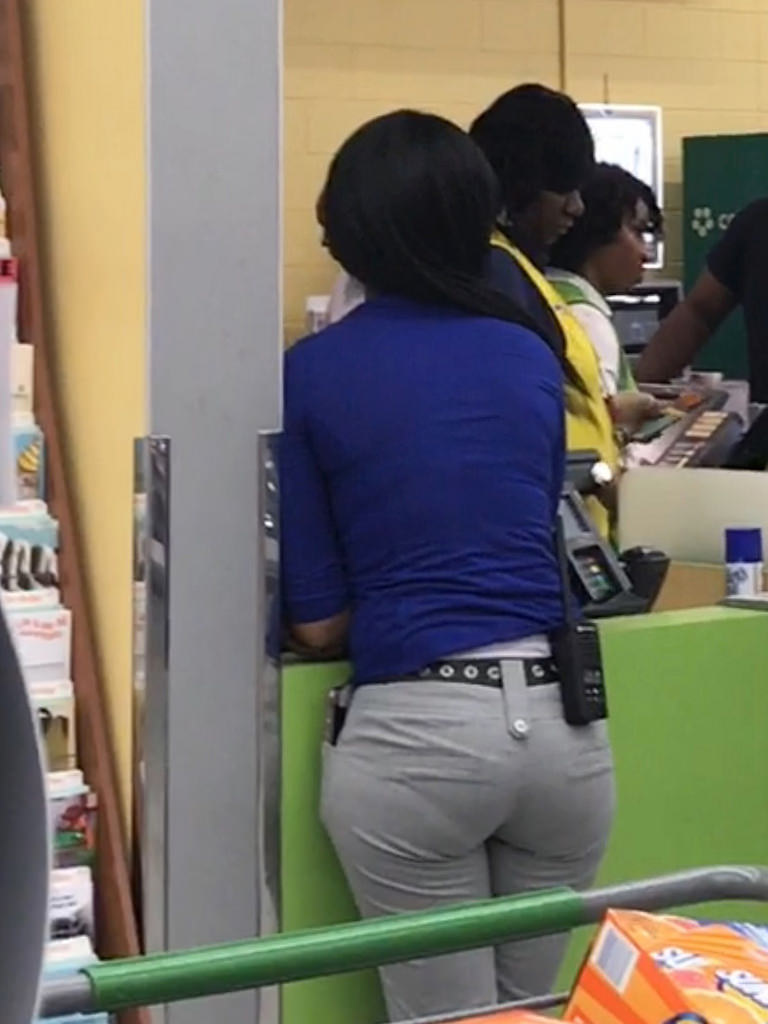In this vibrant, close-up photograph of a grocery store interior, three African American women are prominently featured. Central to the image is a woman facing away from the camera. She has long, dark hair draped over her left shoulder, and wears a short-sleeved blue top with gray pants, accented by a black belt with white studs. A black walkie-talkie is clipped to the back of her belt. She leans slightly against a green counter.

To her right, another woman is visible, dressed in a dark top and green vest, positioned at a cash register. It appears she may be assisting a customer, although the customer, only identifiable by an arm, is cut off from full view.

In the background, against a yellow brick wall, another woman can be seen holding a cell phone, looking towards someone off-camera to the right. Partially visible on the left side of the image is a green and gray cart, which appears to hold a case of soda and brochures peeking out from a shelf. The setting's natural interaction and detailed surroundings heighten the everyday realism of the scene.